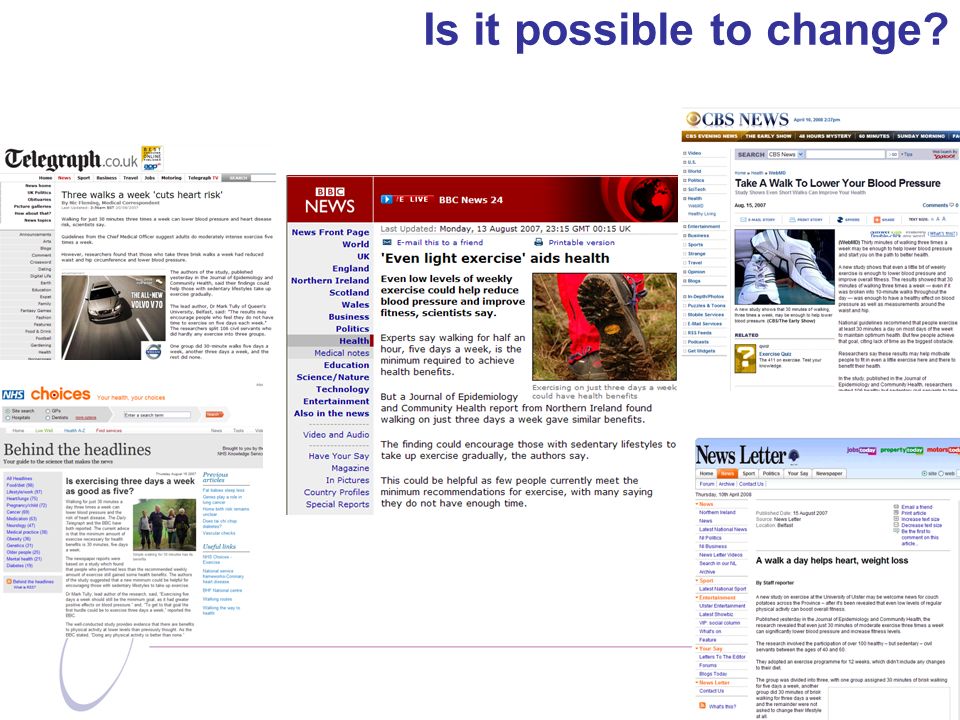A detailed collage designed to promote the benefits of regular exercise. At the top, a bold heading reads, "Is It Possible to Change?"—a poignant question targeting those debating lifestyle changes. The collage features snippets from various reputable sources, each emphasizing the health benefits of walking and other forms of exercise:

1. **The Telegraph**: "Three Walks a Week Cuts Heart Risk"
2. **NHS**: "Is Exercising Three Days a Week as Good as Five?"
3. **BBC News**: "Even Light Exercise Aids Health"
4. **CBS News**: "Take a Walk to Lower Your Blood Pressure"
5. **A Newsletter**: "A Walk a Day Helps Heart, Weight Loss"

Each snippet is rendered on a white background with black text, accented by occasional blue hyperlinks, lending a familiar and credible appearance akin to widely-read online articles. The collage’s format hints at it being something easily shareable on platforms like Facebook, aiming to convince readers that even minimal exercise can offer substantial health benefits.